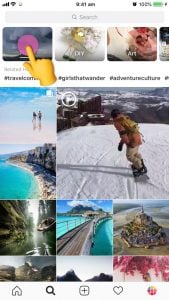A blurry, low-resolution vertical mobile screenshot captured at 9:41 a.m. with a fully charged battery is displayed. The screenshot features a search bar at the top, followed by a series of images. The first indistinct image possibly depicts a gray background with a purple circle and a yellow emoji of a hand pointing at the circle. Adjacent to this image are a white flower on a white background and a pinkish rose labeled "art," next to another image labeled "DIY." Relevant hashtags include #girlsatwinter and #adventureculture.

Below these, the screenshot presents a collection of outdoor-themed images and videos. One notable vertical image shows a vast blue sea curving around cliffs, followed by a video of a snowboarder descending a snowy hill. Additional content includes a river meandering through a lush jungle and a grand bridge spanning a vibrant blue tropical sea, with a picturesque mountainous island nearby.